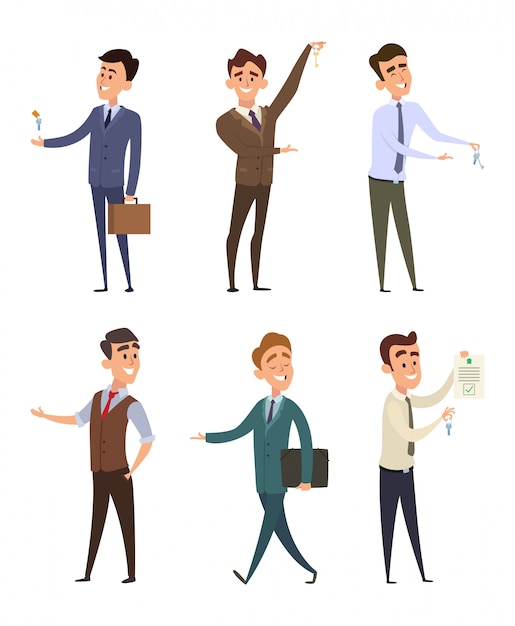The image features six cartoon-like male characters, each with distinct appearances and attires reminiscent of the 1950s or 1960s. All characters are smiling and exhibit upbeat expressions. 

- The top left man has black hair and is dressed in a blue suit. He is tossing his keys into the air.
- The top middle man has dark brown hair and is dressed in a brown suit. He holds his keys as if about to drop them into his right hand.
- The top right man, also with brown hair, is wearing a light blue shirt, blue tie, and black pants. He holds keys in his left hand and is laughing.
- The bottom left man is not holding any keys. He has dark brown hair and is dressed in a light blue shirt, brown vest, red tie, and black pants, smiling broadly.
- The bottom middle man has light brown hair and is smiling so broadly that his eyes are squinted shut. He's wearing a blue suit with matching pants and holds a briefcase in his left hand while gesturing with his right.
- The bottom right man has brown hair and is dressed in a white shirt with blue pants. He holds up a piece of paper with a green check mark and a set of keys, as if about to drop them on the floor.